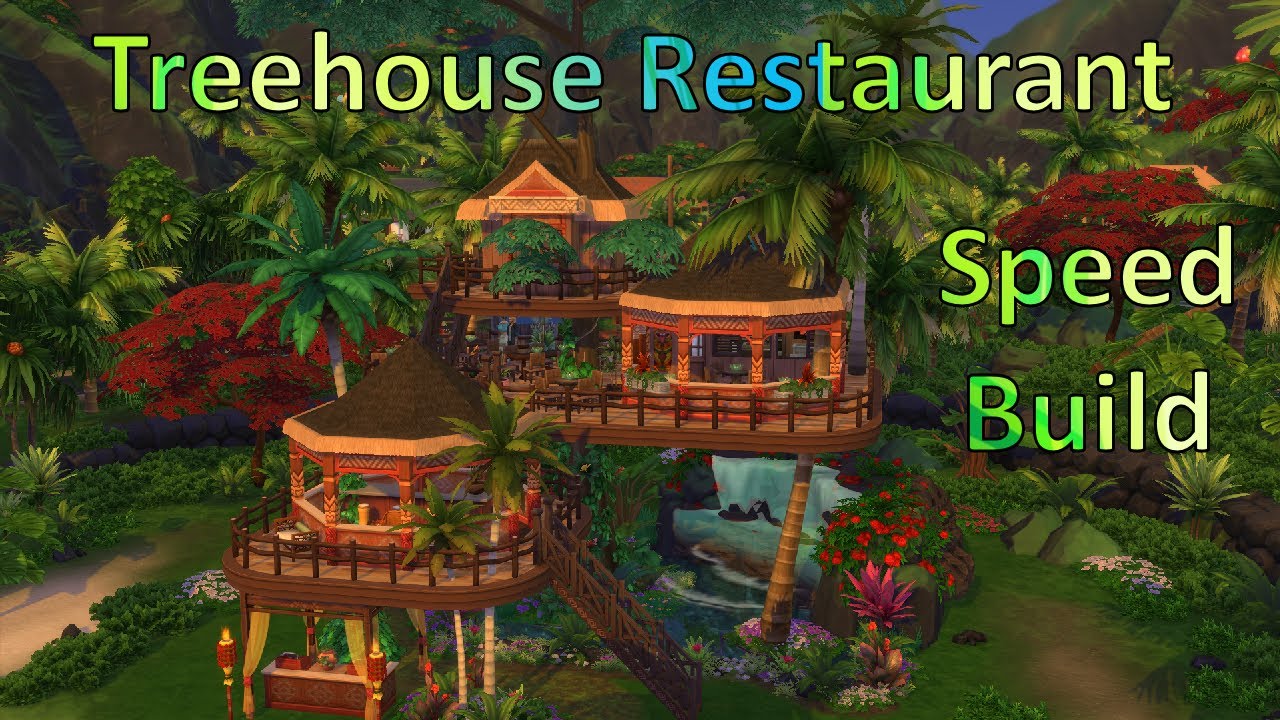This image is a vibrant, 3D-rendered snapshot from a video game, showcasing a lush tropical environment with vivid greenery, colorful flowers, and various hues of reds, yellows, blues, and greens. The scene prominently features a multi-level treehouse restaurant, ingeniously constructed with platforms and stairs that integrate seamlessly with tall palm trees growing through and around the structure. Water flows beneath the treehouse, adding to the serene, natural ambiance. Additional Hawaiian-inspired huts are elevated by coconut trees, set against a backdrop of distant mountains and a waterfall cascading at the center-bottom of the image. Across the top, text in a gradient of lime green, lighter green, and turquoise blue spells out "Treehouse Restaurant Speed Build," emphasizing the playful and creative nature of the setting. This dynamic environment, devoid of people but teeming with life, is reminiscent of a whimsical game landscape, perhaps similar to those found in popular video games like Fortnite.